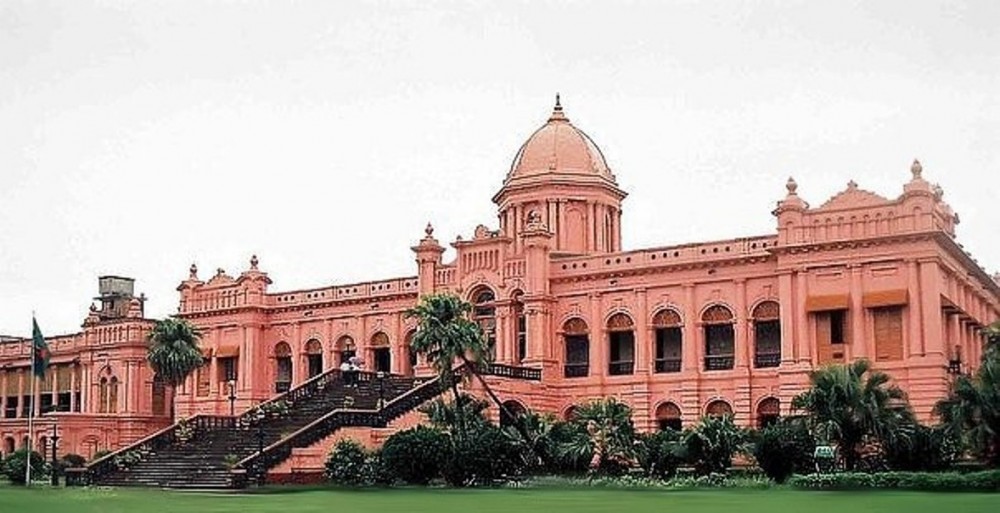This is a color photograph of a large, classical-style building, strikingly rendered in coral pink stone. The building is located in the tropics, as evidenced by the palm trees, shrubs, and small trees in the foreground. The architecture features a cylindrical tower at the center, crowned with a dome-shaped top, and a colonnade of arches leading to a porch. The entrance is accentuated by a long stairway lined with black steps and railings, flanked by outdoor lights. To the far left of the frame, a flagpole flies the flag of Bangladesh—green with a red dot in the center. The building's pink roof extends into the distance on the left, all set against a plain, gray cloudy sky.